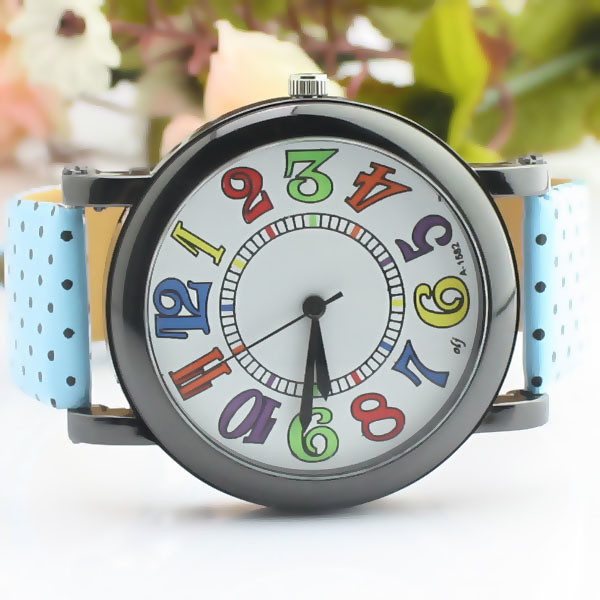This horizontal close-up image prominently features a children’s watch, centered vertically with its bezel and time-setting knob dominating the view. The watch band is light blue adorned with dark, circular spots, adding a playful touch. The bezel is a dark pewter gray, contrasting sharply with the white watch face. The hour, minute, and second hands are all black, offering clear visibility. 

The watch face is decorated with stylized numbers in a colorful sequence: blue at 1 o’clock, yellow at 2, red at 3, green at 4, red at 5, purple at 6, yellow at 7, blue at 8, red at 9, green at 10, purple at 11, and red at 12. Notably, the number positions are unconventional, with 12 located at the center left and 6 at the center right of the face.

Encircling the numbers is a railroad track pattern, matching the color of the adjacent number, adding a whimsical yet educational element to the design. The time displayed on the watch is approximately 8:45.